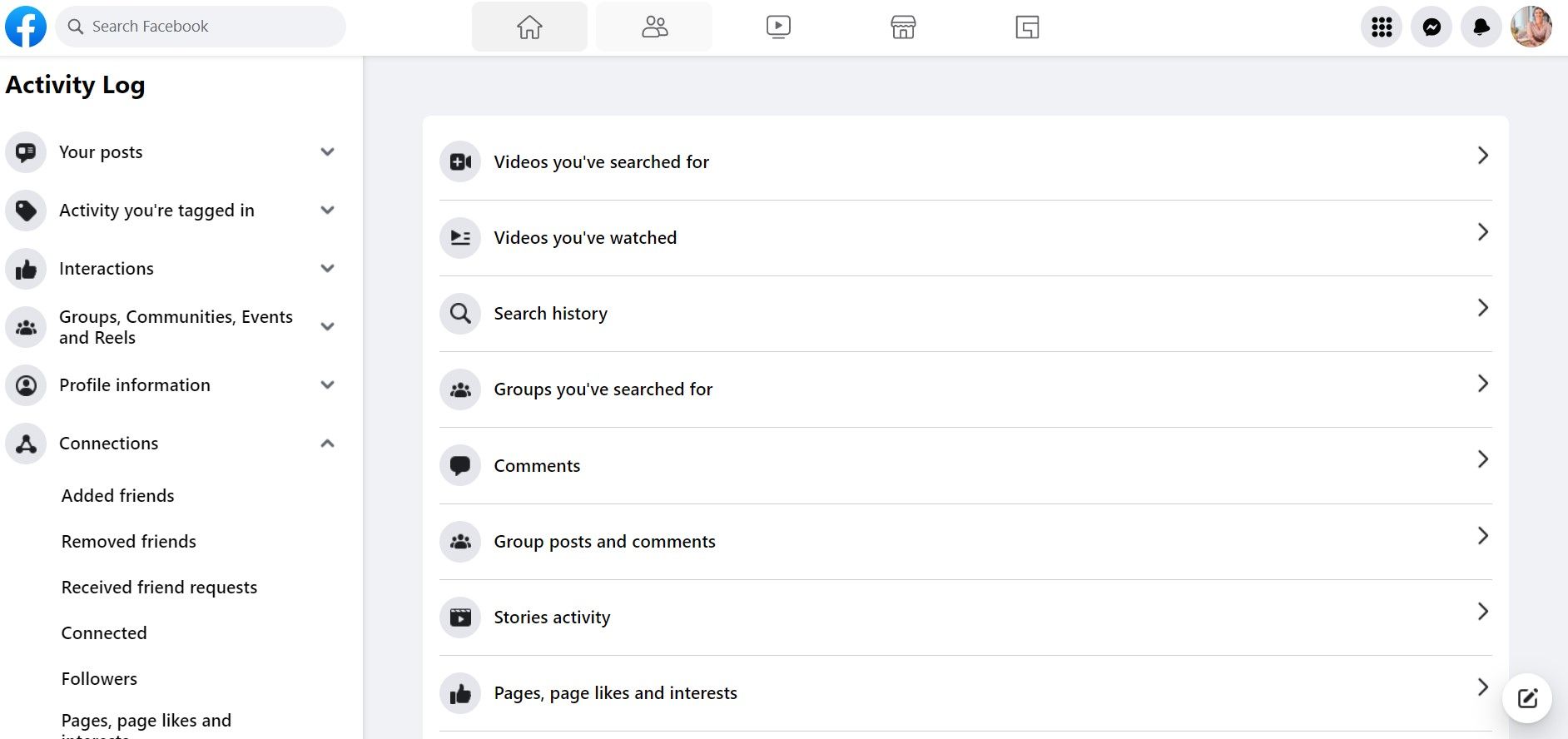This is a screenshot from Facebook's website, meticulously detailed to capture its interface elements. 

At the top, there's a one-inch white border featuring the iconic blue Facebook logo with a white "F" on the left side. Next to it, a rectangular, rounded gray search bar with a black magnifying glass icon and "Search Facebook" text is present. Adjacent to this are icons: a gray background with a home outline, a gray background with an account outline, a play icon, a square with a home icon, and a square featuring a squiggly line resembling a puzzle piece.

On the right side of the border, there's a profile icon displaying a woman with black hair, wearing a long pink sleeve shirt, and seated by a window to her left. To the right of her profile icon, there are icons with gray backgrounds: a black bell (notification icon), a black message icon, and a square composed of three rows of three dots. 

Below this top section, on the left, there's an additional white background featuring "Activity Log" in bolded black text. Underneath it are six icons with corresponding drop-down menus. Below those icons, there are six more clickable items without icons.

To the right of this white background, there’s a lightly gray-bordered area about half an inch thick on the top, left, and right sides. Inside, it contains eight vertical tabs, each with an icon and corresponding text. The first tab has a gray circle with a black video icon next to the text "Videos You've Searched For," followed by a right-facing arrow. There are eight such tabs listed downward.

In the bottom right corner, there’s a small white circle with a black border, resembling a note icon, further enhancing the interface's accessibility and functionality.